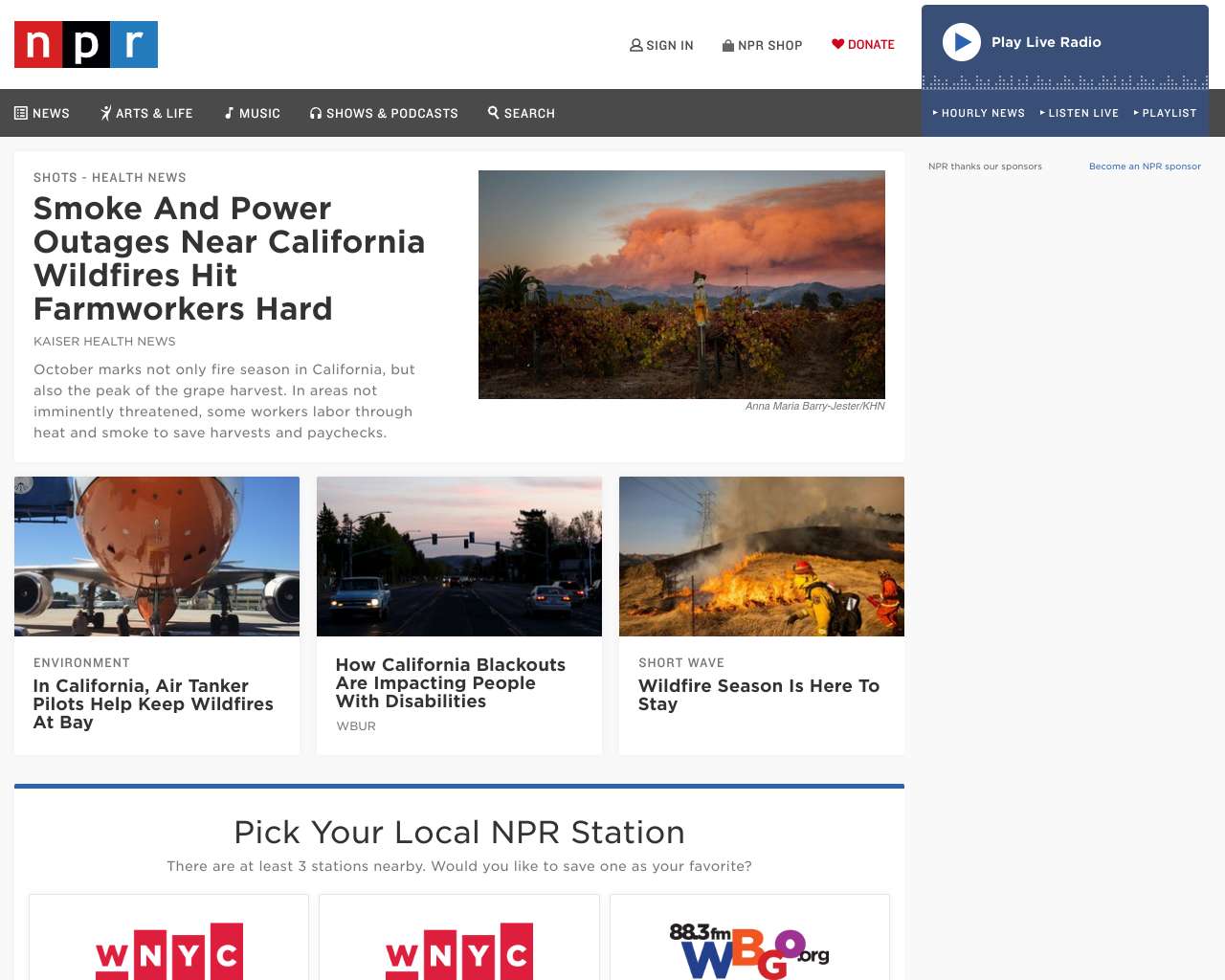The screenshot showcases the homepage of NPR's website. In the upper left corner, the iconic NPR logo is displayed, featuring the letters "NPR" in white within three distinct red, black, and blue boxes. The upper right corner offers several navigation options: "Sign In," "NPR Shop," and "Donate," alongside a blue play button labeled "Play Live Radio."

A horizontal banner spans the width of the page, providing quick links to different sections: "News," "Arts & Life," "Music," "Shows & Podcasts," and a "Search" function.

Just below the banner, a headline in bold reads: "Smoke and power outages near California wildfires hit farm workers hard." This article highlights the dual challenges of fire season and the grape harvest peak in October, detailing how workers toil through extreme conditions to secure their livelihoods.

Beneath this, another headline states: "In California, air tanker pilots help keep wildfires at bay," categorized under the "Environment" section, shedding light on the vital role these pilots play in wildfire management.